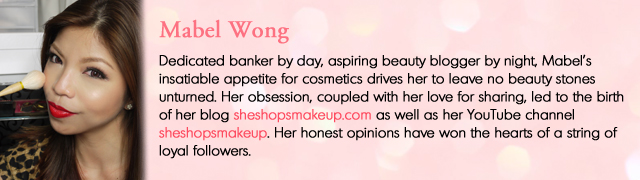This image is a wide photograph with a two-part layout. On the left side, there is a picture of a young Asian woman named Mabel Wong, semi-smiling at the camera while applying makeup to her right cheek with a brush. She has long, dark brown hair with a subtle reddish tint, bright red lipstick, and is dressed in leopard-print attire. The background behind her is whitish-gray. On the right side of the image, against a pink background, is a detailed blurb about Mabel in black text. Her name, "Mabel Wong," is highlighted in pink text. The blurb describes her as a "dedicated banker by day and an aspiring beauty blogger by night." It explains how Mabel's insatiable passion for cosmetics and her love for sharing beauty tips led to the creation of her blog, SheShopsMakeup.com, and her YouTube channel, SheShopsMakeup. Her honest opinions have garnered a loyal following. The links to her blog and YouTube channel are also presented in pink text.